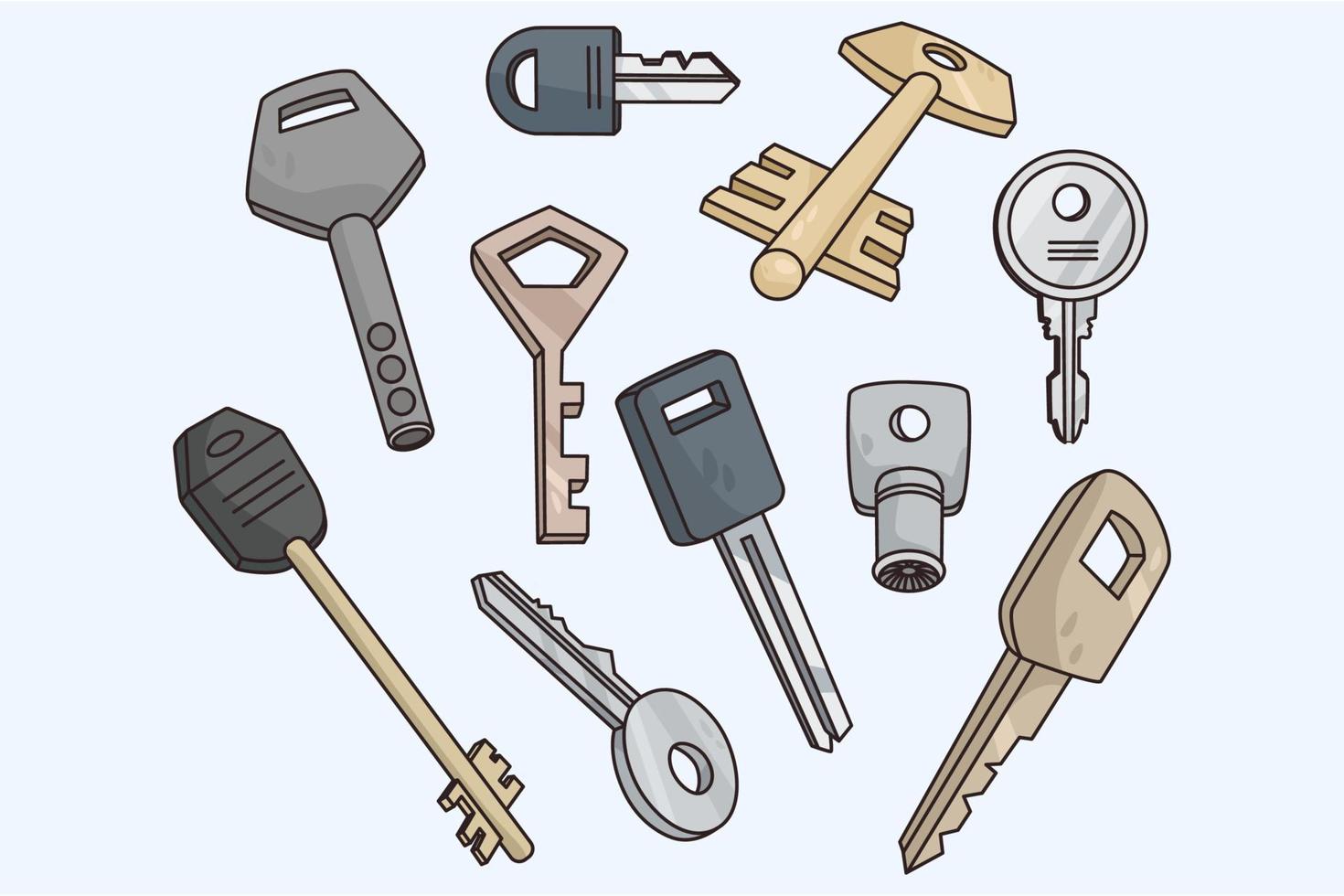This computer illustration features a vibrant, cartoonish depiction of ten assorted keys scattered against a pale blue background. Each key varies in shape, size, and color, showcasing a unique and diverse collection. The keys include shades of gold, brass, silver, and grey, with some featuring black or blue coverings on their heads.

From left to right, the keys exhibit a variety of designs: a key with a black cover and a golden blade with two spikes; followed by a grey key; then a round, silver key; and next, a triangular-topped key in brown. Above these, there's a black-topped key with a silver blade, mirrored below by another black-topped, silver-bladed key. To the upper side is a decorative golden or brass key with old-fashioned wing-like designs, while below it sits an old-style computer key. Moving further right, another round silver key is placed, and underneath lies a brass-colored key resembling a typical house key. 

The precise details in the depiction include keys with multi-tooth blades and different top shapes, such as round, square, oval, and diamond. There is even a key with a unique cylindrical body and circular end, featuring multiple holes, and another key with a distinct small, blue end. This array portrays a rich and eclectic assortment, each potentially fitting into a different lock.